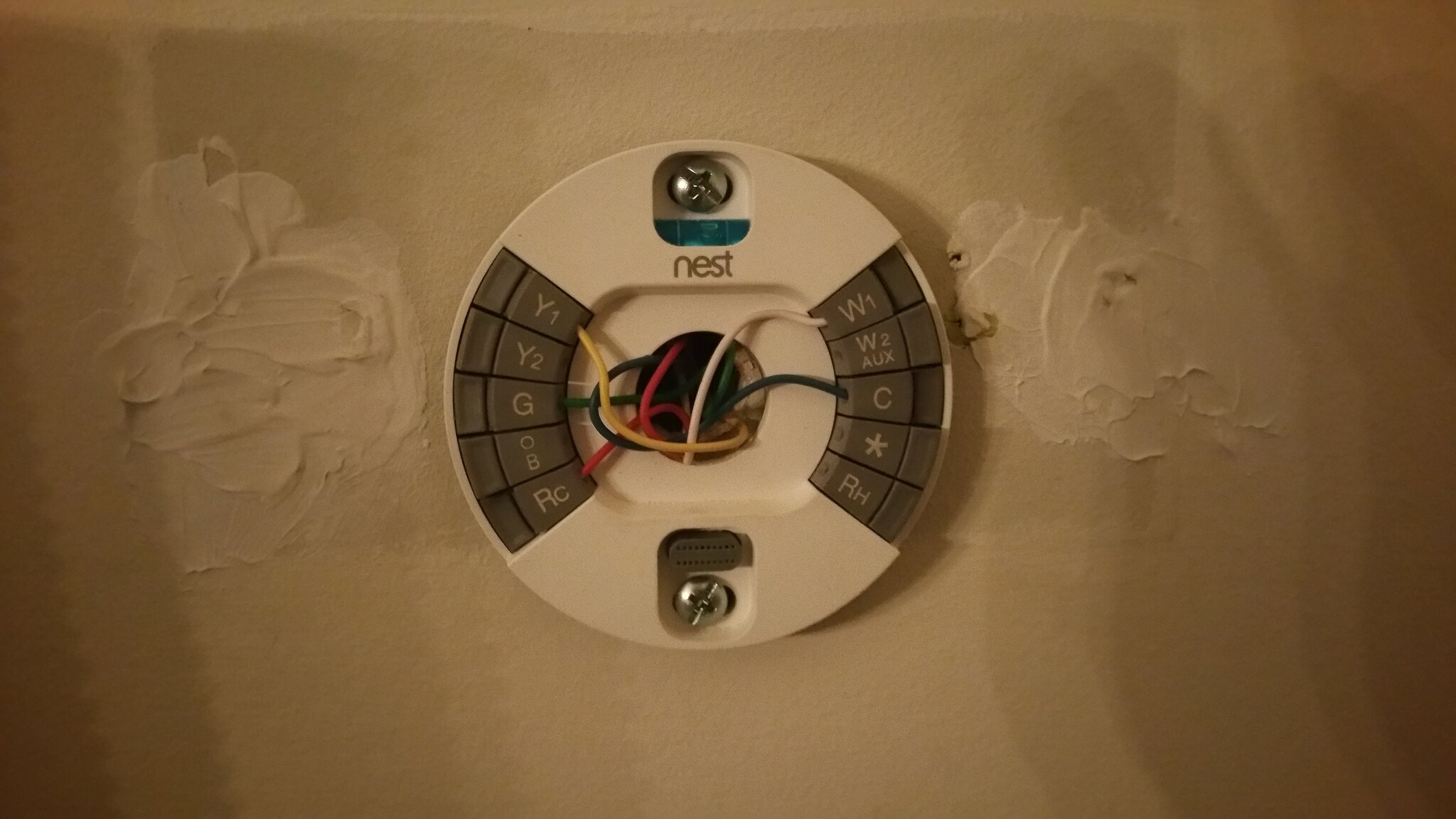A close-up image captures an unfinished white wall with visible repairs. The wall showcases rough, uneven patches where a white filler or drywall mud has been applied, indicating ongoing patchwork. Noticeable are two distinct spots on the left and right sides of the image where the filler has been smeared, resulting in raised, textured areas.

Centrally mounted between these patches is a white plastic component, secured to the wall with silver screws. Emerging from the center hole of this component, and out of the wall, are several wires in various colors: green, yellow, white, red, and black. The plastic piece features gray buttons on both its left and right sides, indicating possible functionality. At the top of this component, just below the upper screw, is a small blue plastic piece. The word "Nest" is imprinted on the white plastic in a grayish or black font, signifying it as a part of the Nest smart home system.